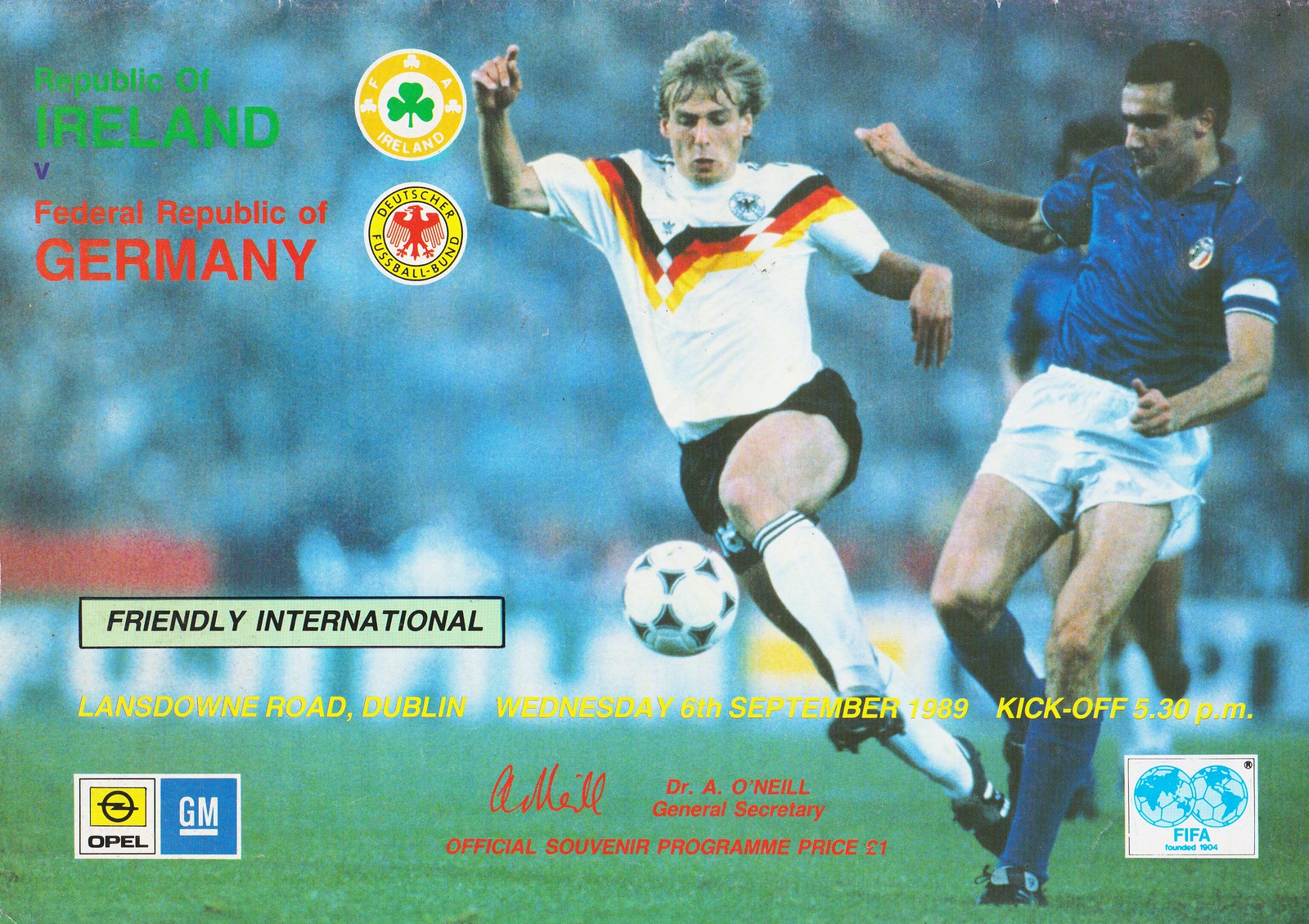This image is an old, grainy, colored poster or flyer for a soccer match between national teams, specifically the Republic of Ireland and the Federal Republic of Germany. The poster features a dynamic scene set in a blurred stadium backdrop with indistinguishable spectators, emphasizing the foreground action. On the right-hand side, a Caucasian player from Germany, wearing a white jersey with black, red, and yellow stripes, black shorts, white socks, and black cleats, is mid-air, preparing to kick a black-and-white soccer ball. Opposing him is a darker-skinned player in a dark blue jersey, white shorts, blue socks, and black cleats, likely of Indian descent, closing in at an angle. Behind them is another player in a similar blue uniform.

In the upper left corner of the poster, in green and red text, are the phrases "Republic of Ireland" and "Federal Republic of Germany" respectively, each accompanied by their national logos. The Irish logo features a yellow-bordered circle with a green three-leaf clover, while the German logo includes a red bird silhouette on a white background with the text "Deutscher Fußball Bund." Below these details, a white bar reads "Friendly International," indicating that the match is an exhibition.

Further down, in yellow text, it specifies "Lansdowne Road, Dublin, Wednesday 6th September 1989, kickoff 5:30 p.m." The lower left corner features two sponsor logos: Opel and GM. Centrally at the bottom, there is a red signature followed by the text "Dr. A. O'Neill, General Secretary, Official Souvenir Program, price one pound." The lower right corner displays the FIFA logo, depicting two joined soccer balls, or globes, in blue, beneath which is written "FIFA."